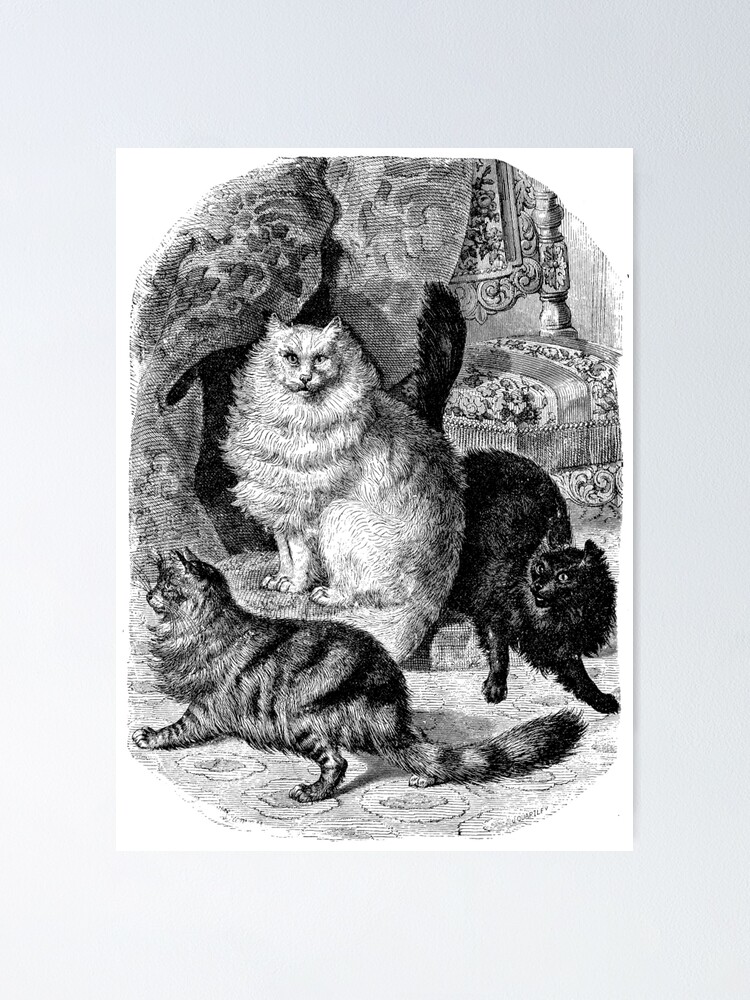The black and white lithograph from the late 1800s or early 1900s intricately depicts three cats gathered indoors, their fine ink lines suggesting a highly detailed pencil drawing. At the bottom left, a striped cat with black and white fur is seen in profile, looking to the left with its tail extended to the right. Above this cat, centrally positioned, a larger white cat with prominent fur on its chest also gazes directly at the viewer, seated gracefully on a cushion. To the right, a fully black cat, its body angled to the right but head turned left, appears to be stepping down from a raised surface like a cushion, with its tail held straight up. This indoor setting hints at a cozy, possibly historic living space adorned with fabric drapes showcasing intricate patterns, and floral-patterned rugs underfoot. In the background, a bed with scrollwork on its post and intricately patterned fabric hangs, evoking an old-world charm, potentially symbolizing early domestication scenes of cats.